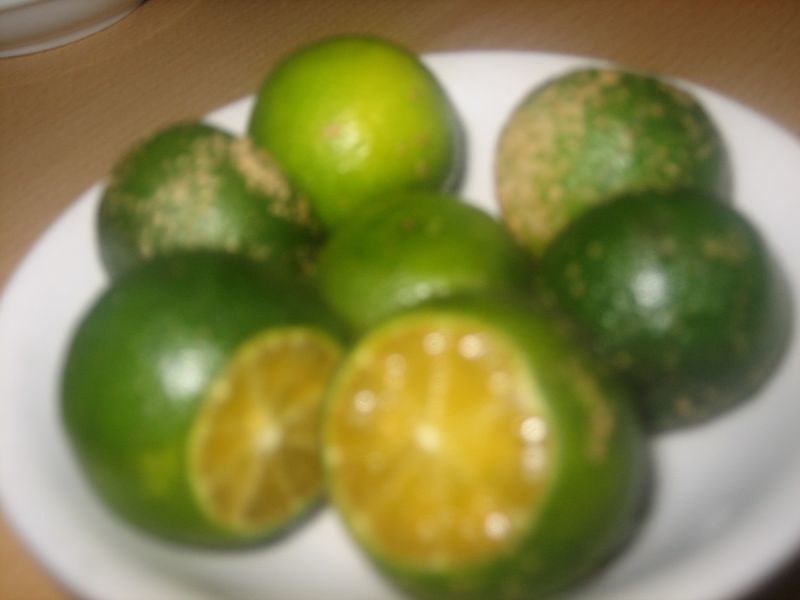This image features a close-up, albeit out-of-focus, view of a white round dish holding seven green citrus fruits identified as Citrus Madurensis, commonly known in Malaysia as Limau Kasturi. The fruits, which resemble small limes roughly the size of slightly larger golf balls, are positioned closely together. Two of these fruits have their ends sliced off, revealing their partitioned, slightly yellowish-green interiors. The rinds of some citrus fruits exhibit brown discoloration and white speckles, possibly indicating natural variations or mold. This white dish rests on a wooden table surface, with another plate or bowl faintly visible in the background.